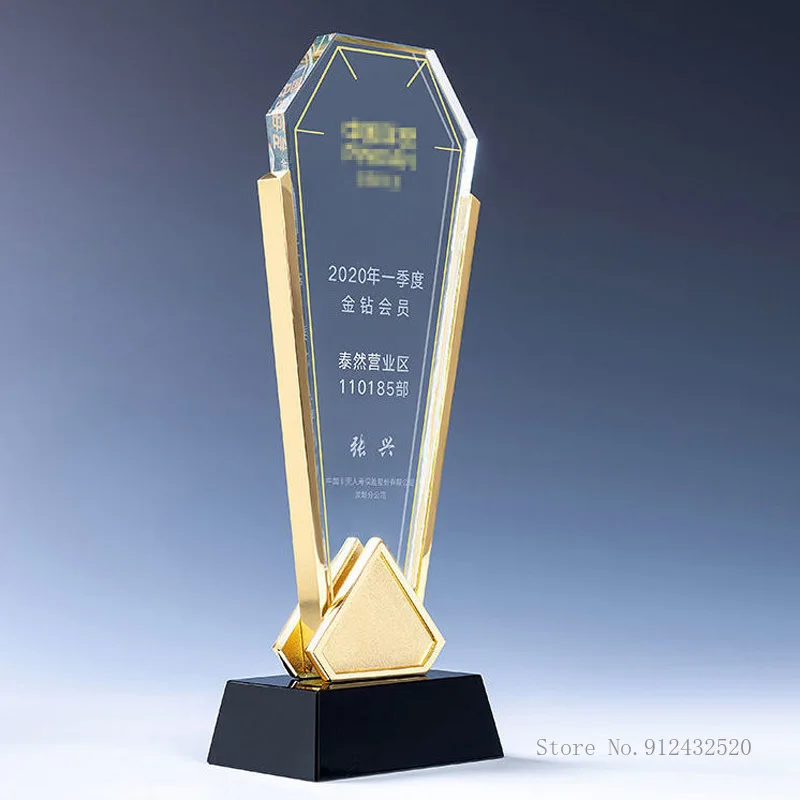This image features a striking award trophy with a unique design. The trophy is mounted on a black wooden-like base, with a gleaming gold triangular element at the center that extends into elegantly shaped gold arms. These arms frame a clear, crystal-like surface that is meticulously engraved with text. The text includes the year "2020" and additional characters that appear to be in an Asian language, possibly Chinese or Japanese. The background of the image is a gradient that transitions from dark blue in the upper right corner to a lighter blue or white in the bottom left, creating a visually appealing contrast. A series of numbers, "110185," is also visible on the award, likely denoting specific details or achievements. In the bottom right corner of the photo, English text reads "store number 912432520," indicating the recipient or relevant store for the award.